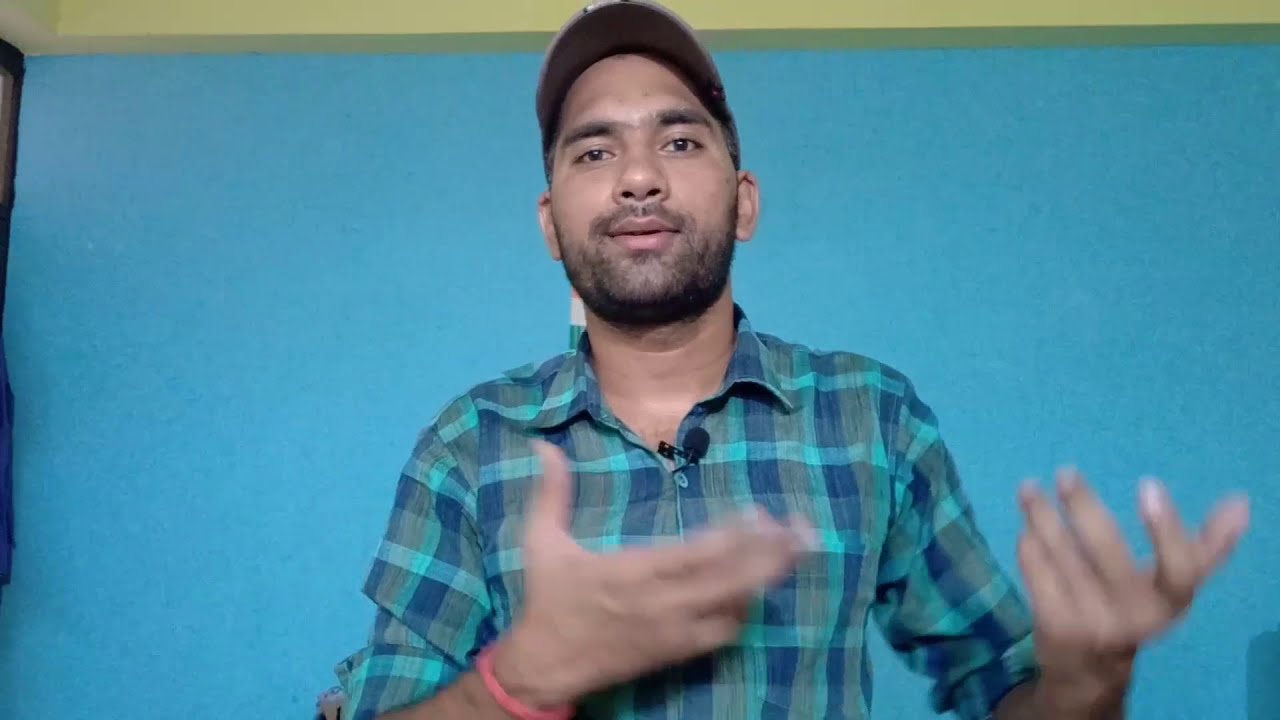In this horizontally oriented image, we see a young man, possibly of Indian or Middle Eastern descent, standing in front of a blue backdrop that appears to be a projector screen. A white band at the top suggests either a wall or the mechanism from which the screen is pulled down. The man is dark-skinned, wearing a blue and green plaid button-down shirt with an open collar through which a professional lavalier microphone is clipped. His attire includes long sleeves, and he sports a dark beard and a baseball cap. 

He's animated, gesturing with both hands—his right hand (on our left) is raised over his chest and somewhat blurry from motion, indicating he's mid-speech, possibly making an emphatic point. His left hand (on our right) is also slightly blurred, positioned off to his side. Noteworthy is the pink or orangish bracelet adorning his right wrist. The scene looks like a screen grab from a video, set in a generic room with a hint of a light greenish-yellow ceiling. The overall ambiance and his focused gaze into the camera enhance the impression that he is delivering a lecture or a presentation.